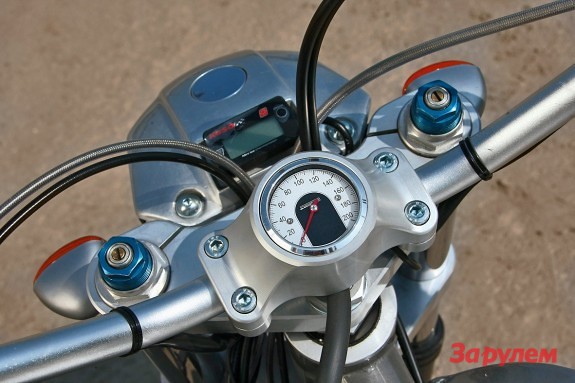This photograph features the front view of a two-wheeled vehicle, likely a smaller motorcycle or possibly an electronic scooter. The vehicle appears to be a dirt bike, judging by its compact and rugged design. The handlebars are prominently visible, equipped with a speedometer that measures speed in either miles per hour or kilometers per hour. Two distinctive royal blue bolts are noticeable on the front, complementing the light blue or silver detailing of the bike’s facade. 

Multiple wires, comprising two black and two silver, extend towards the front section, possibly serving various electronic and mechanical functions. The vehicle is also adorned with red lights or reflectors on the front, contributing to its visibility and safety. Additionally, a black tube runs from the top downward, potentially part of the vehicle's steering or suspension system.

Despite its scooter-like appearance, indicated by the commenter’s uncertainty about its classification, the high speedometer range suggests it might indeed be a motorcycle. In the bottom right-hand corner of the image, the text "3APYNEM" is legibly inscribed. Overall, the vehicle's hybrid features — between a motorcycle and an electronic scooter — make it a unique mode of transportation.